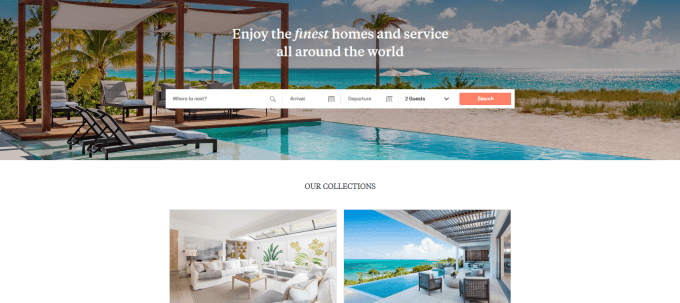The advertisement showcases luxurious vacation destinations and high-end hotel accommodations with a vibrant, scenic image spanning from left to right. The top half of the image captures a serene blue sky with scattered clouds. Below the sky lies a picturesque blue ocean stretching across the entire width of the frame. Near the center, two small white barges are visible, with three more to the right. The left side features lush palm trees and a manicured grassy area that transitions into a sandy expanse with two shaded lounge areas. Each lounge is covered by a white tarp supported by four brown poles and accompanied by light brown outdoor chairs. The scene is complemented by a sparkling blue pool at the bottom of the image, with two additional chairs on a concrete surface in the left corner.

Overlaying this idyllic scene, text in white reads: "Enjoy the Finest Homes and Service," followed by a second line stating, "All Around the World." Below this, a white search bar stretches halfway across the page from the middle, offering a tool for finding such exquisite experiences. 

In the lower portion of the advertisement, the section titled "Our Collections" showcases two inset images. The first inset, located to the left, depicts an elegant hotel room with a white couch, gray cushions, and white walls adorned with floral patterns. The room features brown flooring, adding a touch of warmth to the space. The second inset, on the right, introduces a stunning balcony view. From the left, the image reveals a broad expanse of sky with some clouds, a glimpse of the sea, a tree line, a pool, and a concrete area furnished with two brown chairs and a brown table. This detailed scene encapsulates the luxury and sophistication promoted by the advertisement.